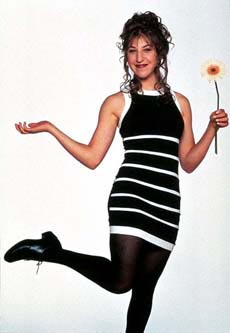In this small, slightly blurry, vertically rectangular photograph approximately 1.75 inches wide by 2.5 inches high, the actress Mayim Bialik is captured in a distinctive pose against a plain white, slightly hazy background. Bialik, with her light skin and brown, curly hair styled up with wispy side pieces and bangs, is smiling gently. She is wearing a form-fitting, off-the-shoulder mini dress that is black with thin, horizontal white stripes. The dress has a subtle, broader stripe just above the mid-thigh and a white trim at the top. Matching her sophisticated outfit, she has on black shoes with small heels and black stockings. Bialik's left hand extends outward, holding a yellow and white gerbera daisy, while her right hand is raised to the side with her palm facing up. Her right leg is bent at the knee, lifting her foot slightly off the ground, adding a dynamic element to her poised stance.